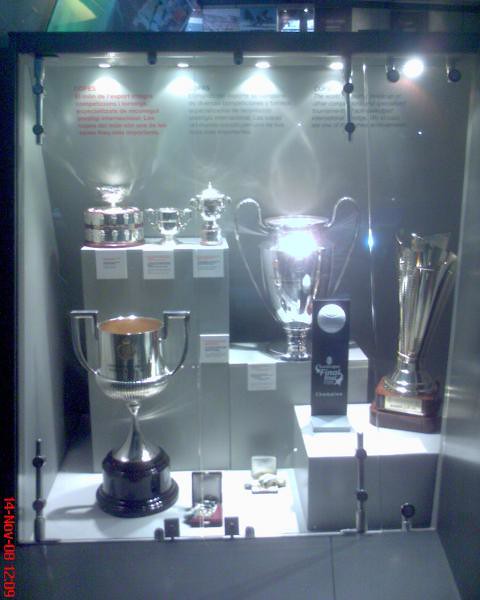This color photograph features a sophisticated indoor trophy case with a dark metal border and illuminated interior. The front of the case is glass, allowing a clear view of the numerous trophies displayed inside. Overhead and interior lighting enhances the visibility of the trophies, causing a reflective glare that gives them a bright shimmer. The trophies are arranged neatly on several shelves and podiums within the case.

On the left side stands the tallest and largest trophy, which is gold with a substantial base. Adjacent to it, on a prominent rectangular podium, is a larger trophy with two handles on the sides. The top rectangular shelf houses three smaller, hand-sized trophies, while a smaller cube podium in the front displays two additional mid-sized trophies. Another notable item is a narrow black rectangular box situated horizontally, showcasing a white ball on its top. All trophies are accompanied by white square labels with descriptive text, albeit too small to read. This exquisitely lit and organized display mimics what one might expect to see in a museum or sports hall of fame.